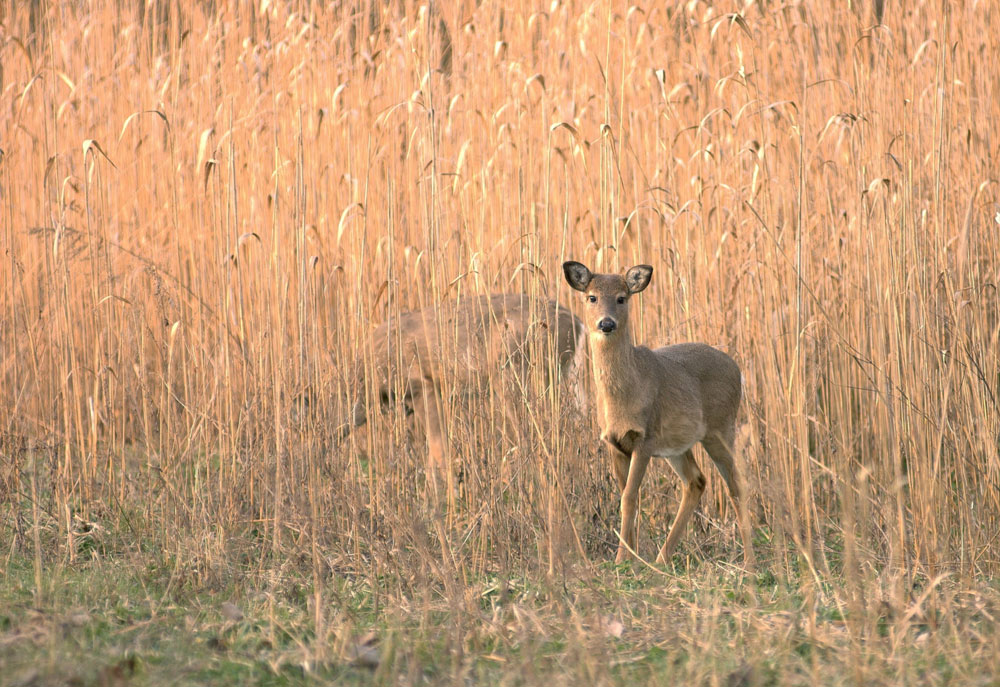A captivating photograph captures a young deer standing tall and alert in the wild, surrounded by a sea of golden, dried-out stalks that resemble a mix of wheat and possibly corn. The focal point of the image is the deer, positioned toward the center, gazing directly at the photographer with its expressive, black eyes. Its coat is primarily light brown with patches of black fur on its chest and white fur on its belly. The deer's erect ears, darker on the outside and white on the inside, hint at its attentiveness. The scene suggests a fall setting, with the tall brown stalks towering above the green grass interspersed beneath. The deer's black nose and the detailed texture of its fur add to the vividness of the image. In the backdrop, blending almost seamlessly into the golden foliage, another deer, possibly younger, with its head down as if grazing, adds depth to the tranquil and picturesque scene likely captured at dawn or sunset, bathed in a soft, golden glow.